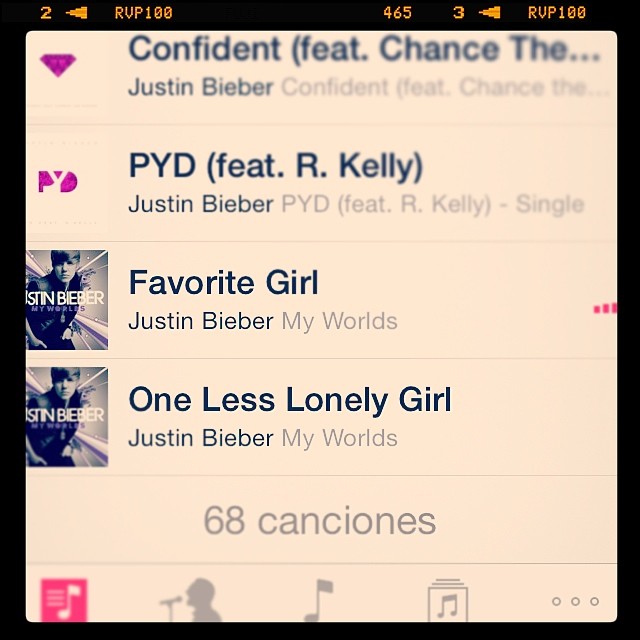The image is a screenshot from a music app displayed on either a smartphone or computer screen, framed by a black border and set against a pink background. At the top left corner, there's a label that says "2" next to a left-facing triangle, followed by the text "RVP 100". On the top right, the text "465 3 RVP 100" is visible, each with a left-facing triangle nearby. Below these top labels, the screen is divided into multiple horizontal sections, each containing music-related information.

The first section features a song titled "Confident" by Justin Bieber, with a pink diamond icon. The second section lists "PYD" featuring R. Kelly, followed by Justin Bieber’s initials. The third and fourth sections contain tracks "Favorite Girl" and "One Less Lonely Girl," both credited to Justin Bieber from the album "My Worlds." Further down, there is an indication of 68 songs ("68 CANCIONES").

At the bottom of the screen, four distinctive icons are observed including a set of three dots in the right-hand corner, which is likely for accessing additional options. Avatars and text are spread across the screen with musical symbols appearing next to song titles, reinforcing the theme of music selection.